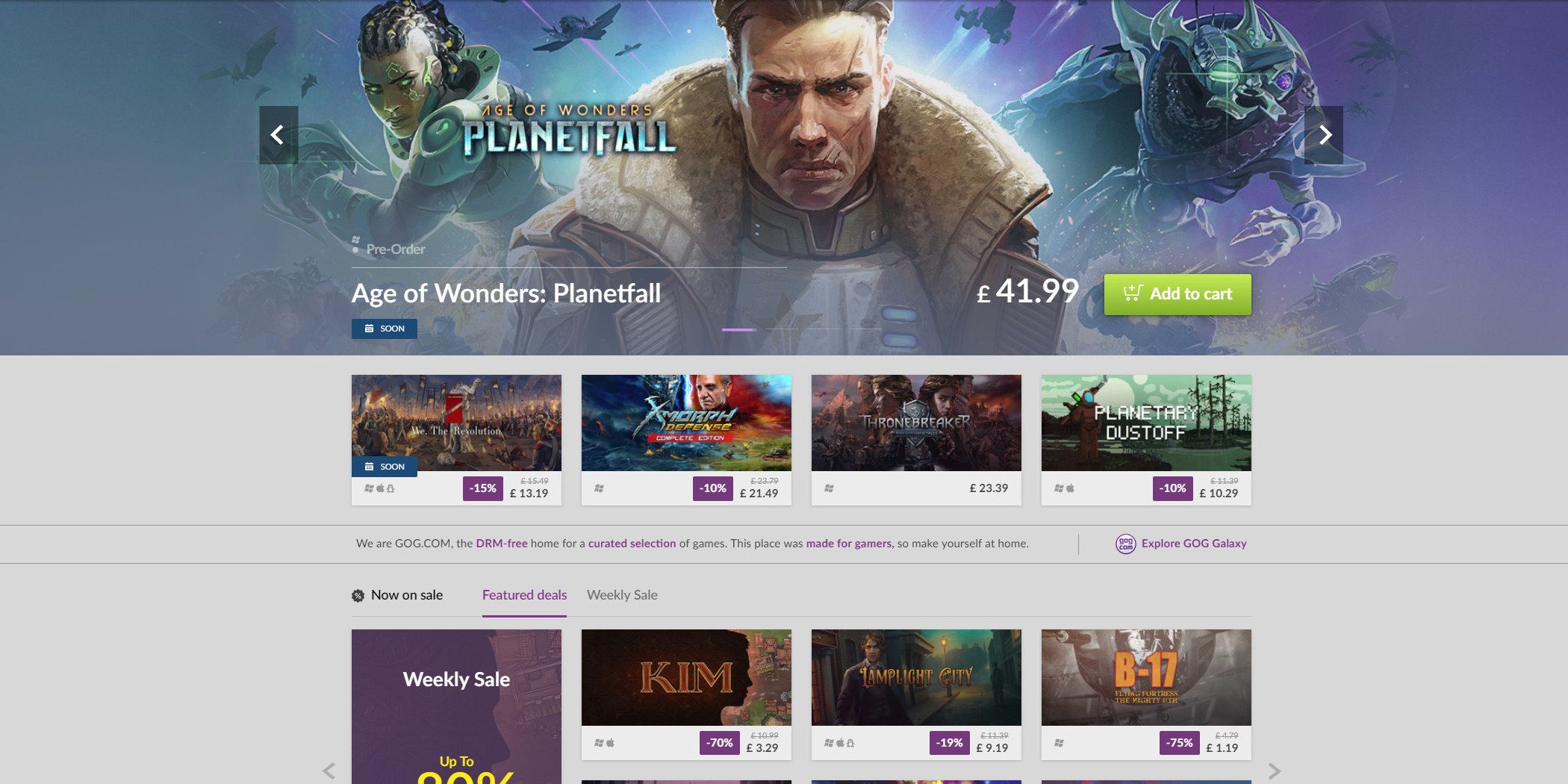The image depicts a website showcasing various game listings. At the forefront is an illustration for the game "Age of Wonders: Planetfall." The central figure is a man with distinctive facial scars and a large, fluffy collar on his jacket. To his left, a woman is depicted in a spacesuit, while to his right stands an alien being. The background features numerous ships set against a purplish-blue, space-themed backdrop. The title "Age of Wonders: Planetfall" is prominently displayed in white text below the illustration, along with the price of £41.99. Below this, there is a green "Add to Cart" button.

Under the main game listing, several other game thumbnails are visible. Although the title of the last game is unclear, other games like "Morph Defense," "Thronebreaker," and "Planetary Dustoff" are listed. The section also features a tagline for the website: "We are GOG.com, the DRM-free home for a curated selection of games. This place was made for games; make yourself at home." Further down are more game icons, including titles like "Kim," "Lamplighted City," and "B-17." Additionally, there is a mention of a weekly sale on the left side of the page.